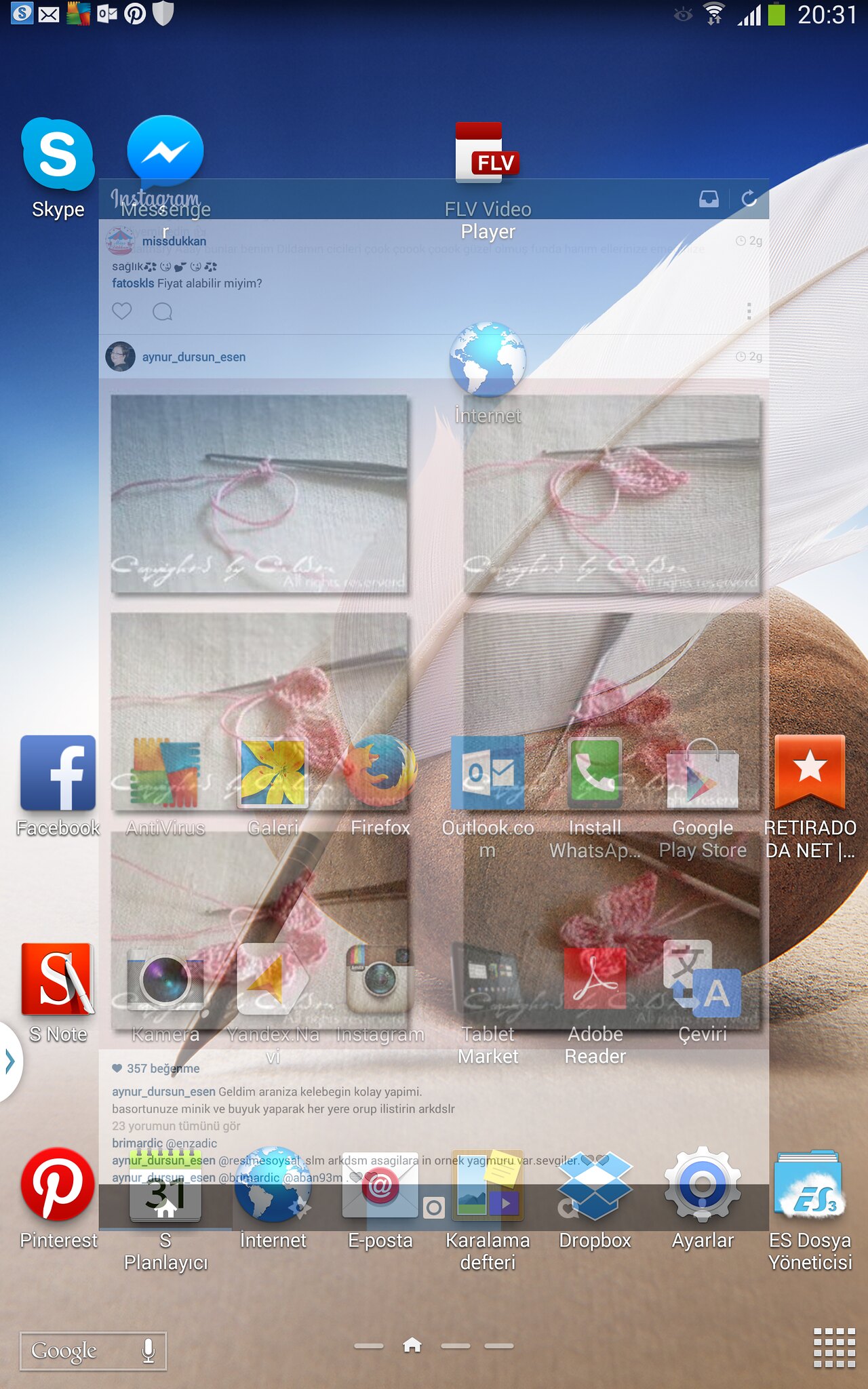This image displays a detailed screenshot of what appears to be a tablet home screen with a user interface typical of an Android device. The screen prominently features a blue background adorned with a white feather and pink strings, alongside a subtle image of a coconut and quill feather. At the top of the screen, the status bar shows a green battery icon, four signal bars, a two-bar Wi-Fi icon, and the time, which reads either 2031 or 2081. 

The main screen is populated with an array of commonly used app icons such as Facebook, Pinterest, Dropbox, Skype, Instagram, Messenger, Plan IEC, Internet, e-poster, and more. Notably, a floating, transparent overlay displaying Instagram is open in the center of the screen, partially obscuring other elements. Additionally, at the bottom of the screen, there is a home button, with a "Google" label in white on the bottom left and more app icons including Pinterest on the bottom right. The screenshot captures a typical busy home screen, reflecting a mixture of social media, communication, and productivity apps.